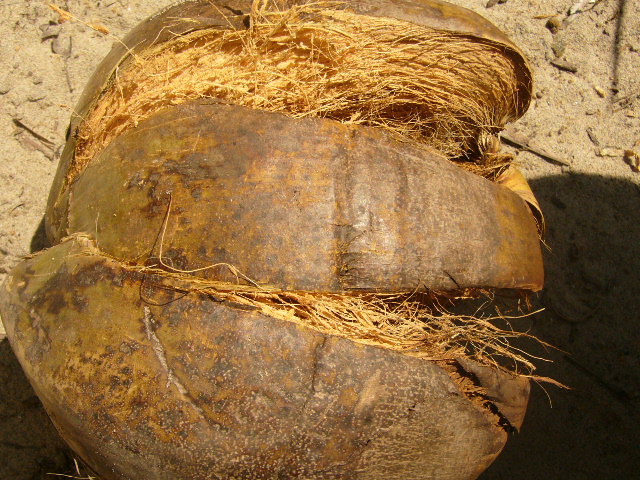The image depicts a large, brown object resembling a dried, split-open coconut, resting on a brown, rocky terrain. The object's exterior is rough and husk-like, indicating age and decay, while its interior comprises fibrous material similar to hay or straw. The coconut-like object is distinctly divided into two sections, revealing the fibrous content within. Surrounding it is a ground that appears sandy and earthy, scattered with small rocks, twigs, and wood chips. The scene casts a shadow on the lower part of the image, enhancing the earthy, organic tones of brown, orange, and yellow. Despite uncertainty about its exact nature, the object strongly resembles an old, rotten coconut with visible brown spots and fibrous material spilling from its openings.